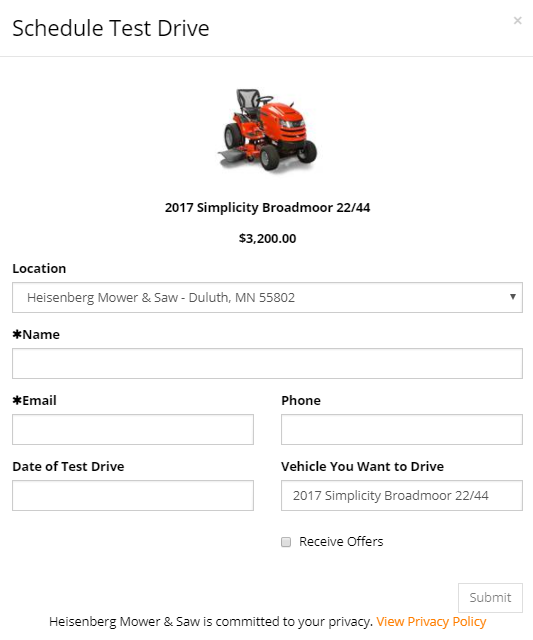The screenshot displays a mobile app interface for Heisenberg Mower and Saw, specifically a menu for scheduling a test drive. The featured product is the 2017 Simplicity Broadmoor 22/44, accompanied by a thumbnail image. The cost of this mower is listed as $3,200 USD.

The interface contains several fields required to schedule the test drive. Users must provide their name and email, both marked as mandatory fields with an asterisk. Additionally, fields are available for entering the desired test drive date and the user's phone number. The vehicle information, "2017 Simplicity Broadmoor 22/44," is auto-filled to the right of the date selection box.

An optional checkbox is visible, allowing users to opt-in for receiving offers. At the bottom, a privacy policy notice assures users of Heisenberg Mower and Saw's commitment to privacy, with a clickable link to view the full policy. The "Submit" button is currently inactive, indicating that the required fields have not yet been completed. 

The location for the test drive is specified as Heisenberg Mower and Saw in Duluth, Minnesota, with the postal code 55802.